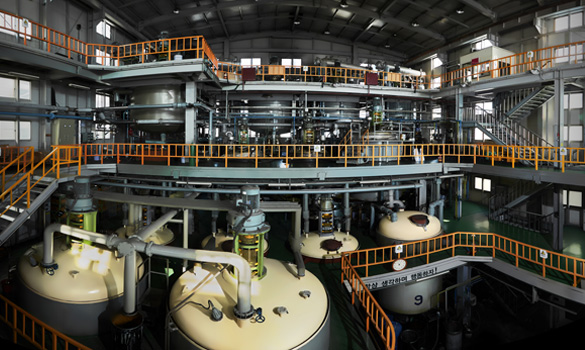This photograph captures the inside of a multi-level industrial facility or factory, likely housed within a warehouse. The image, taken with a wide lens, reveals at least three observable floors, each safeguarded by bright orange safety railings which stand out against the otherwise cold, metallic, gray environment. The bottom floor features several large cylindrical vats interconnected by numerous pipes, suggesting the presence of complex industrial processes. Stairways on the side provide access to each level. Higher floors are equipped with various machinery and additional piping, indicating a highly mechanized space. On the bottom level, there is also some text in Japanese or Korean, adding a regional context to the setting.